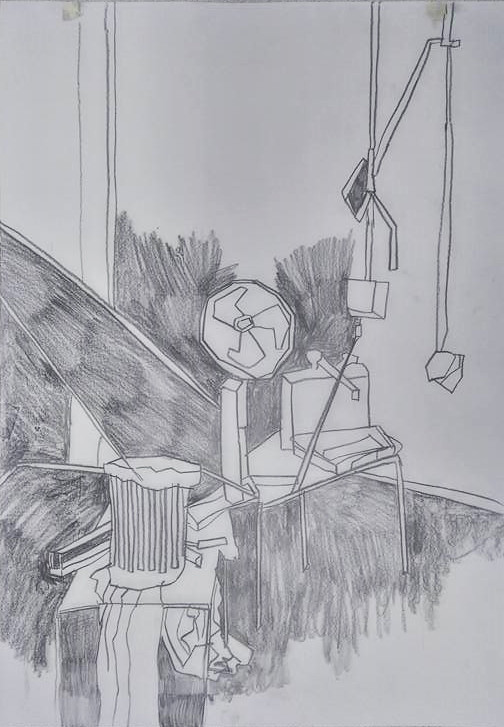This meticulously hand-drawn pencil illustration intricately captures the ambiance of a cluttered workspace. In the bottom left corner, a small dresser is visible, viewed from the side, making its exact form slightly ambiguous. Atop the dresser sits a container resembling a trash bin, with various objects spilling out haphazardly. Dominating the scene is a desk featuring a rectangular item whose purpose is unclear, possibly a device or appliance. Nearby, a stand is topped with what appears to be a fan, though its design raises concerns due to its uncanny resemblance to a controversial symbol. The flooring around the desk and sections above it are heavily shaded in dark gray, adding depth and contrast to the composition. Suspended from the ceiling are several microphones, lending a sense of activity and focus to the workspace. The artist's attention to detail and shading accentuates the chaotic yet intriguing nature of the scene.